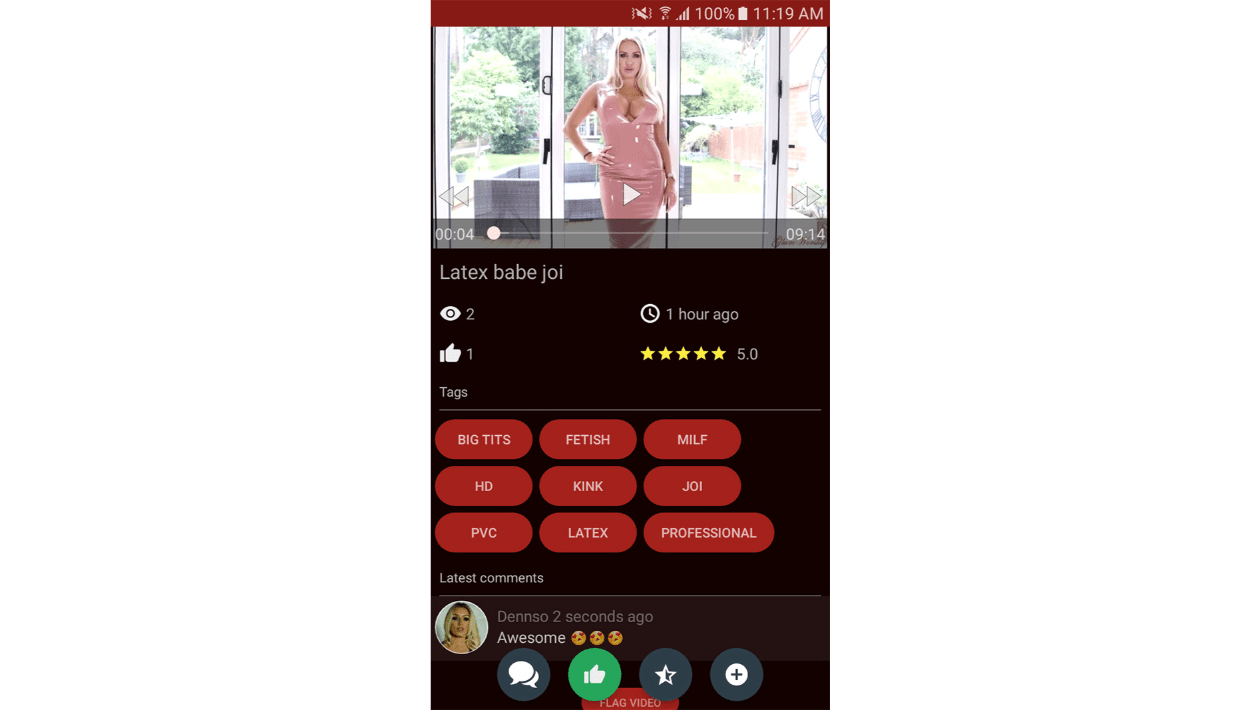Screenshot of a phone displaying a video thumbnail captioned "Latex Babe Joy." The thumbnail features a woman posing with one hand on her hip in front of large glass folding doors, revealing a backyard with a clothes hanger, outdoor seating area, and several trees. She is dressed in a revealing, tightly-fitted pink dress. The video, posted one hour ago, is nine minutes long and has received a thumbs up, been viewed twice, and has a five-star rating. Numerous tags related to the video indicate its pornographic nature. At the bottom of the screen, a comment made two seconds ago by a user with a profile picture reads "awesome," accompanied by three like emojis.